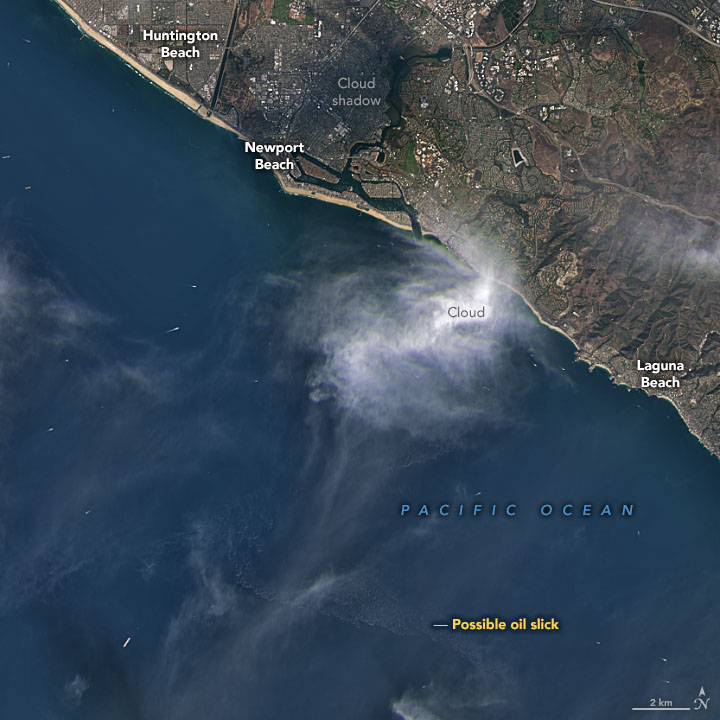This image is a detailed aerial photograph of the Pacific Ocean along California's coast. The ocean, a striking blue, occupies the bottom left two-thirds of the image, while the land stretches diagonally from the upper left to the right third of the photograph. Notable coastal cities such as Huntington Beach, Newport Beach, and Laguna Beach are marked along this stretch of land. A cloud is beginning to hover over the shore, casting distinct shadows on the green and brown-toned terrain below. The land reveals small details like houses, streets, and undulating mountains, albeit very tiny from this high altitude. Additionally, there is a labeled "possible oil slick" area in yellow notation toward the bottom of the image, indicating a suspicious patch in the water. The photograph includes a scale marker indicating a distance of two kilometers and an arrow pointing north, providing orientation for the viewer.